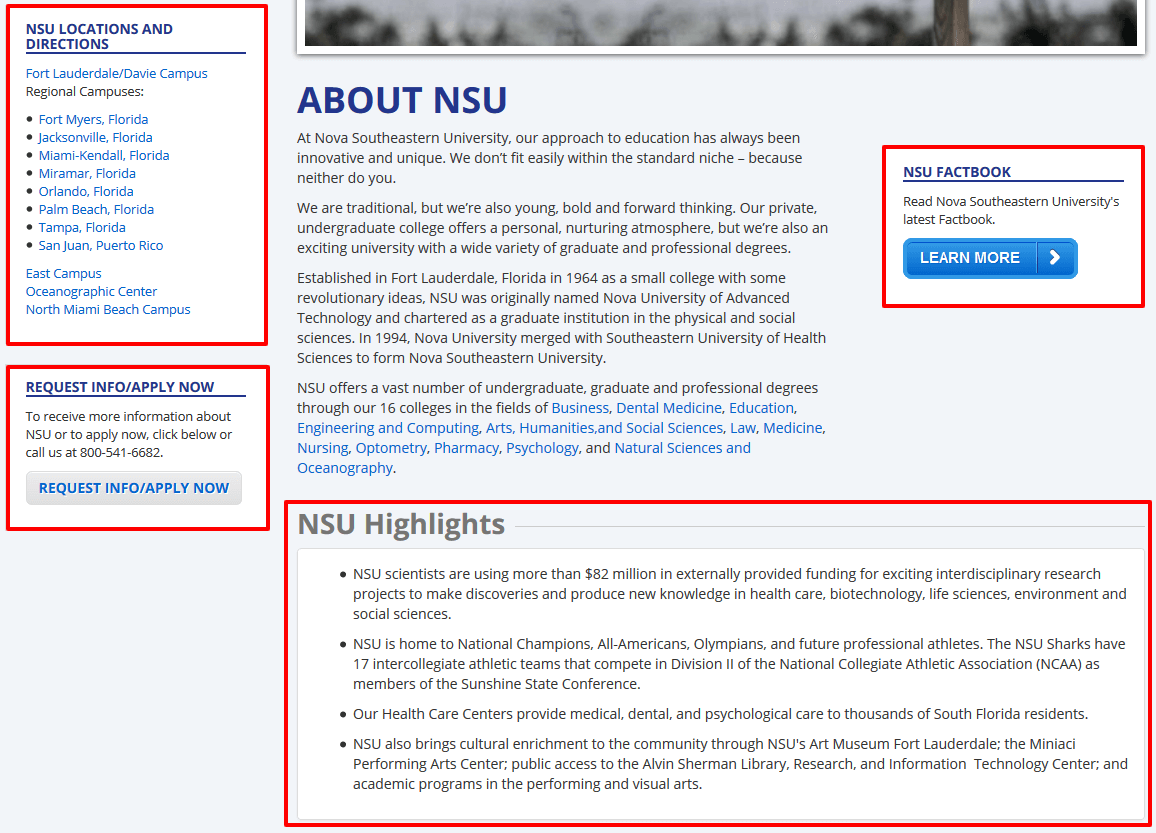A screenshot from the Nova Southeastern University (NSU) website is shown. The top-right and center portion of the screenshot shows the edge of a blurry black and white photo, the details of which are unclear. In the upper left-hand corner, there is a text box with a red band superimposed on it, listing NSU locations and directions. The listed locations include Fort Lauderdale campus, regional campuses across Florida, a campus in Puerto Rico, East Campus, North Miami Beach, and the Oceanography Centre.

Below this section, another red-outlined box is visible, containing options to "Request Info" or "Apply Now." This section invites users to click for more information about NSU or to apply, offering a button for "Request Info" and "Apply Now" and providing a call number.

To the right of this, a larger block of text is dedicated to details "About NSU." The text emphasizes the innovative and unique approach to education at Nova Southeastern University, claiming that they don’t fit easily into the standard niche, reflecting the individuality of their audience. 

At the bottom of this block, a list of faculties is written in blue. Adjacent to this, on the right side of the screenshot, is a segment titled "NSU Factbook," inviting users to read the latest facts about NSU through a blue button outlined in red.

At the very bottom of the screenshot, there's a section titled "Highlights," also outlined in red. This section includes several bullet points highlighting various aspects of NSU such as their Olympians, funding, healthcare centre, and cultural environment.

Overall, almost every element on the website is emphasized by red outlines, drawing attention to important features and options for prospective students and visitors.